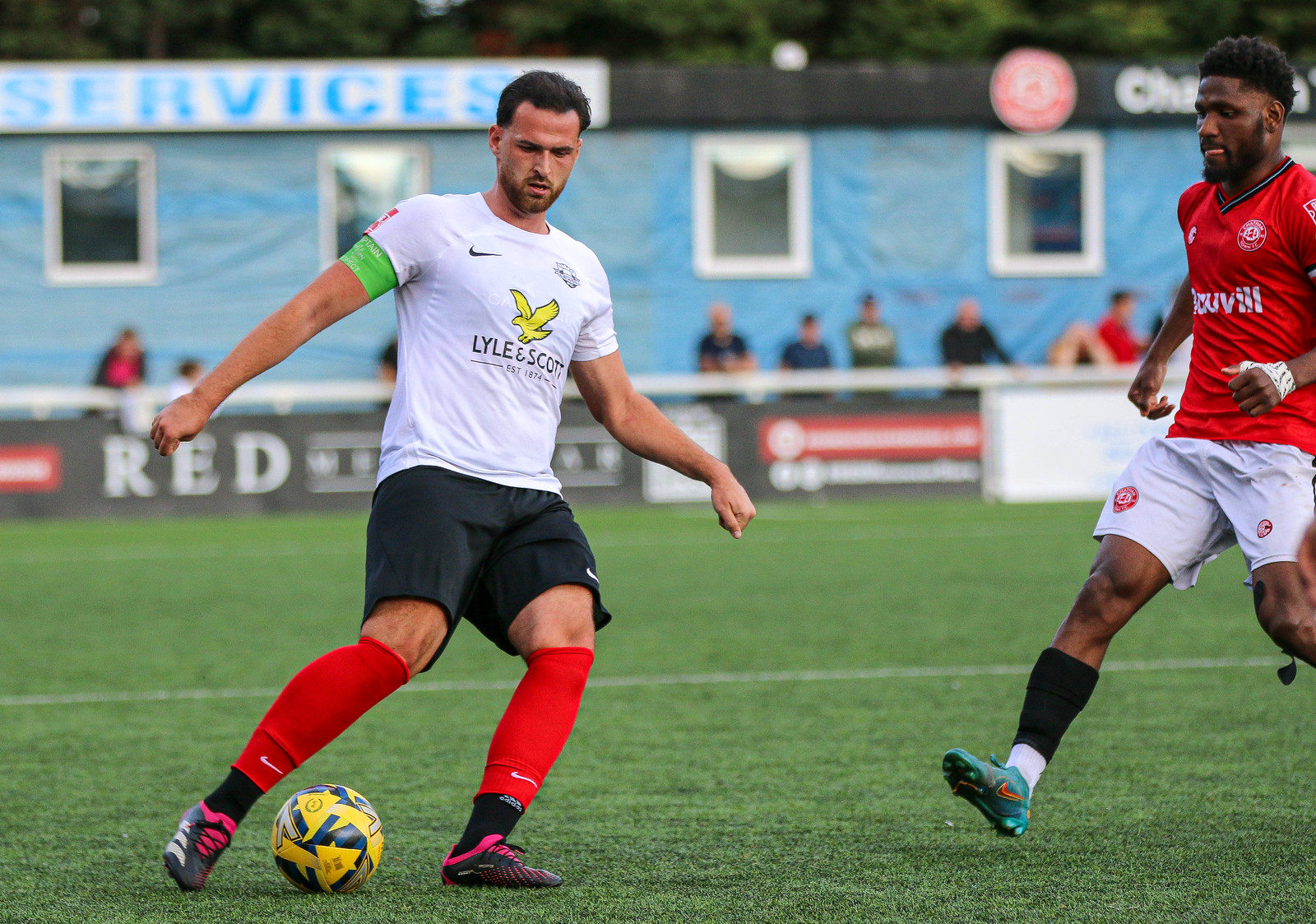In this photograph of a soccer game, two men are shown on a bright green field with a faint yellow-white line behind them. The man on the left, wearing a white short-sleeved jersey with "Lyle and Scott" printed on it and a gold-colored eagle emblem, is poised to kick a yellow, blue, and black soccer ball positioned close to his foot. He is dressed in black shorts, red socks with a Nike emblem, and black shoes with pink stripes. The man on the right, a black man with black curly hair, a full beard, and mustache, is running towards the ball with his tongue sticking out in concentration. He wears a red jersey, light gray shorts, black socks, a white brace on his hand and thumb, and light blue Nike shoes, one of which is tilted with toes up, showing he is standing on his heel. The background is blurry, revealing people behind a barrier, a white square sign with "Services" on a blue background in the upper left corner, a mostly blue building with white-framed windows, and a black banner with red and white text. A red box with white text is also visible on the left side of the banner.